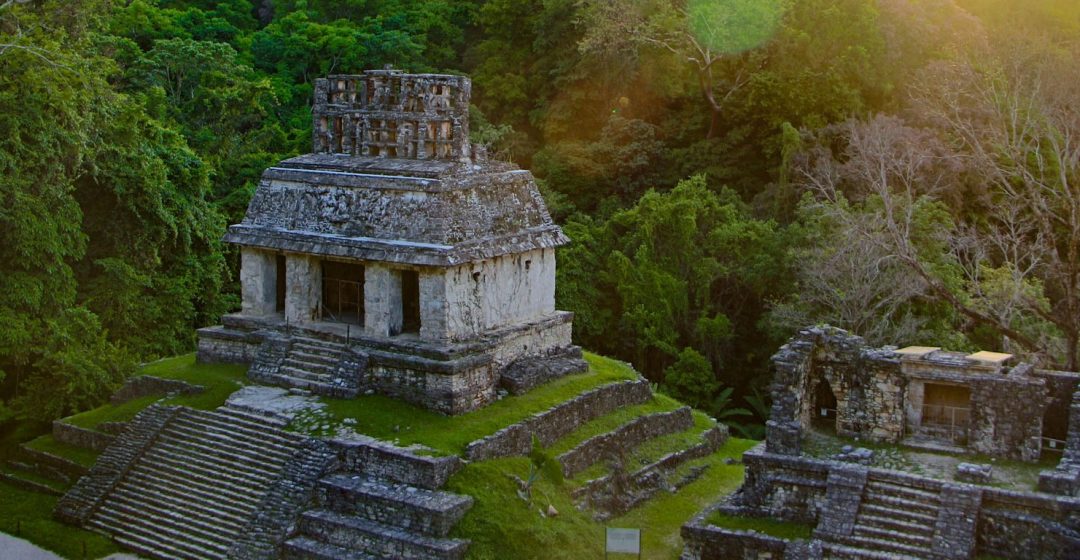The image depicts ancient Mayan ruins, likely situated in a lush Mexican jungle. The greenery is dense, with massive trees enveloping the scene and grass growing on the structures. Central to the image is a rectangular temple sitting on a terraced hill, featuring steps that lead to its summit and then to its entrance. This main building exhibits significant wear, with missing chunks of its exterior and decorative elements on the roof. 

Adjacent to the main structure, on the right, stands another, more dilapidated building with partially standing walls and an absent roof. Both structures are made of stone, weathered by time, with moss and vines overtaking them, underscoring their ancient origins. Various grates and retaining walls attempt to flatten the terraced ground around the temple, enhancing its grandeur. The overall scene is a captivating blend of human history and the relentless encroachment of nature.